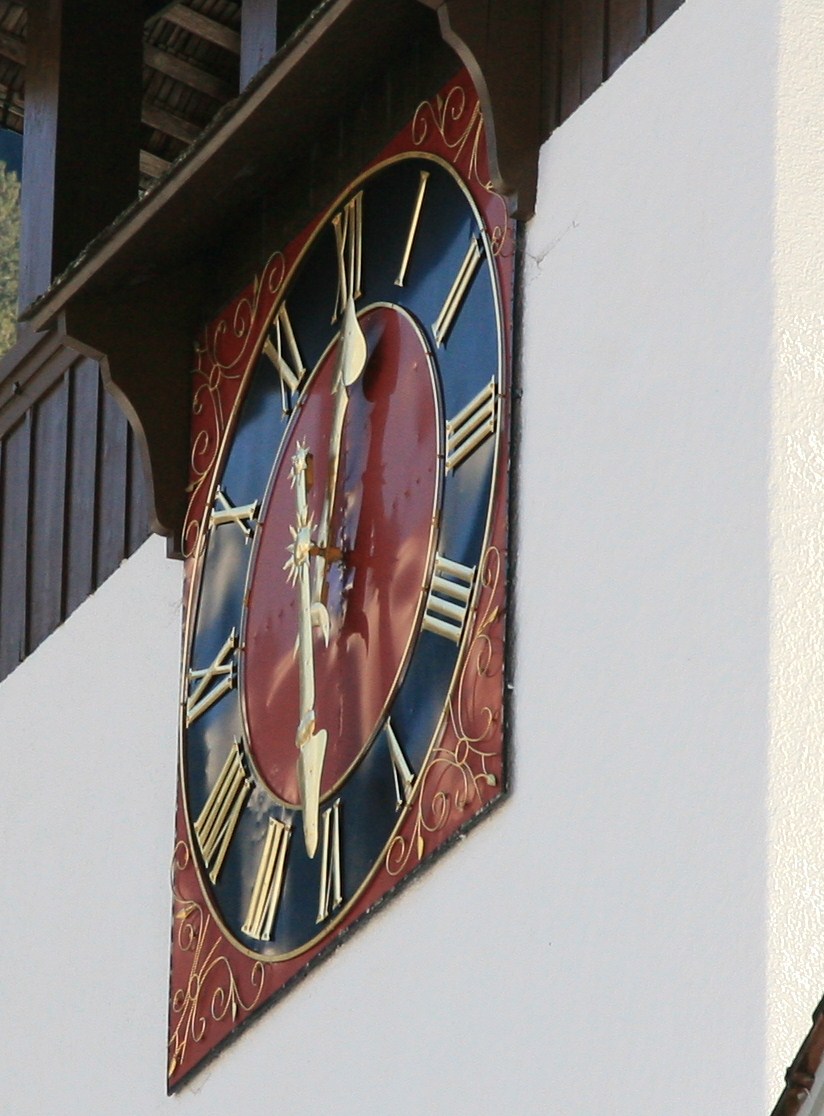The image captures a large, ornate clock mounted on a white facade of a two-story building. The clock, positioned just above the first floor, features a rectangular maroon backplate adorned with gold filigree designs. Its round face is marked by gold Roman numerals and large, gold hands displaying the time as 12:30. The clock face includes a shiny, burgundy center with a sun face on the hour hand, and a black outer ring containing the numerals. Above the clock, a brown wooden shelf extends, casting a shadow over the top. The building's wall includes a lower section painted white and an upper section made of wood. This section is framed by dark brown beams and posts, resembling a gazebo structure. From the ground level vantage point, the clock appears to be an integral part of an elaborate overhanging facade, complete with a balcony and roof beams.